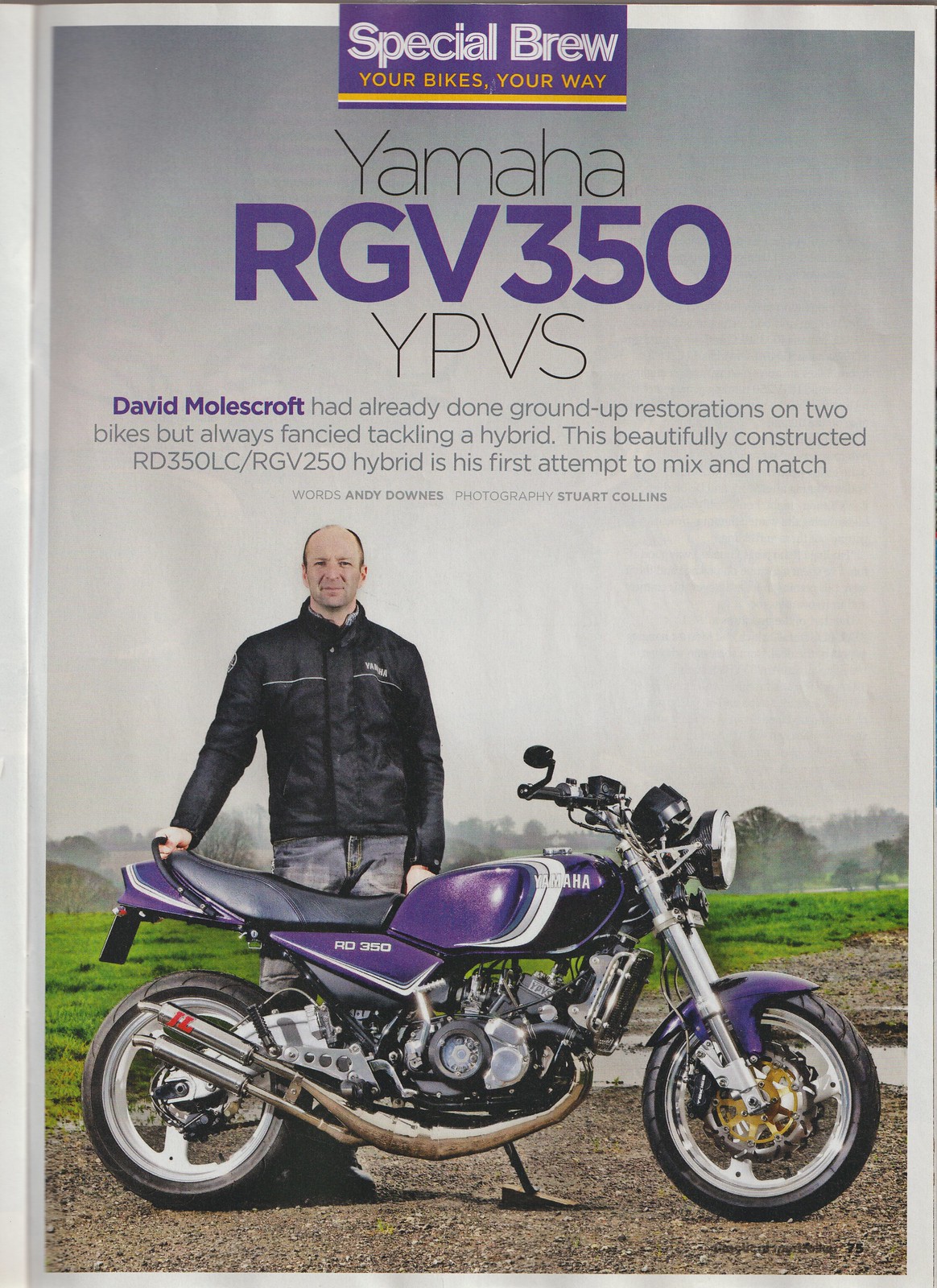In this image, we see David Molescroft, a bald man wearing a black leather jacket and jeans, proudly standing behind his meticulously restored purple Yamaha RGV350 YPVS motorcycle. His bike, a stunning RD350LC/RGV250 hybrid blend, features a black seat, black handlebars, a silver engine with a silver front fork, gold calipers, and red exhaust wrapping. The background shows a mix of grass, trees, and some rocky terrain, enhancing the sense of an outdoor setting. The photo, which seems like a vintage advertisement or magazine cover, prominently displays the headline "Special Brew" in white font against a purple backdrop, followed by the slogan "Your Bikes Your Way" in yellow. David's achievement in creating this unique motorcycle gets highlighted with a caption detailing his journey of mixing and matching bike parts, underlining his first successful hybrid project.